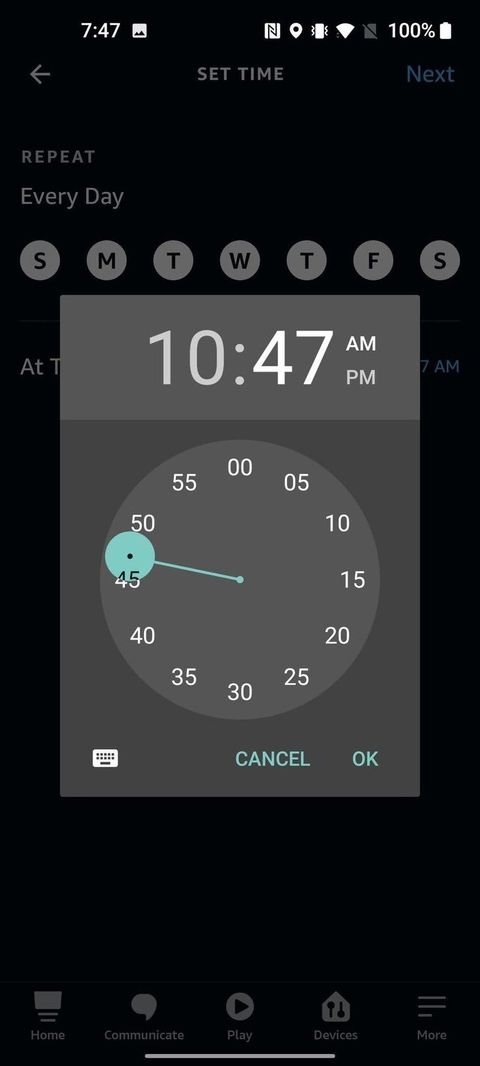This image is a screenshot taken from a smartphone showing the interface for setting the time. The background color is black, specifically at the top left corner. At the top of the screen, the time is displayed as "7:47." To the right of the time, there is a white battery icon indicating that the battery is fully charged at 100%. Next to the battery icon, the Wi-Fi signal icon is visible, along with an icon that indicates the phone is set to mute.

Beneath this status bar, gray text on a black background reads "Set Time," confirming that this is the screen used to adjust the device's time settings. In the center of the screen, a gray rectangular box displays the current time set at "10:47," with the "AM" option selected.

Directly below the displayed time, there is a circular clock interface for adjusting minutes and possibly seconds, marked at intervals such as "00," "05," "10," "15," and so on. At the bottom right corner within the gray box, there are two buttons labeled "Cancel" and "OK," allowing the user to either discard the changes or confirm the new time setting.

Outside of the gray box but still within the black background, on the left side, the text "Every Day" is shown, followed by a sequence of gray circles each containing a letter representing the days of the week: "S," "M," "T," "W," "T," "F," "S" (Sunday through Saturday).

At the very bottom of the image, the footer of the phone's interface is visible, displaying various standard icons commonly found on a smartphone's navigation bar.